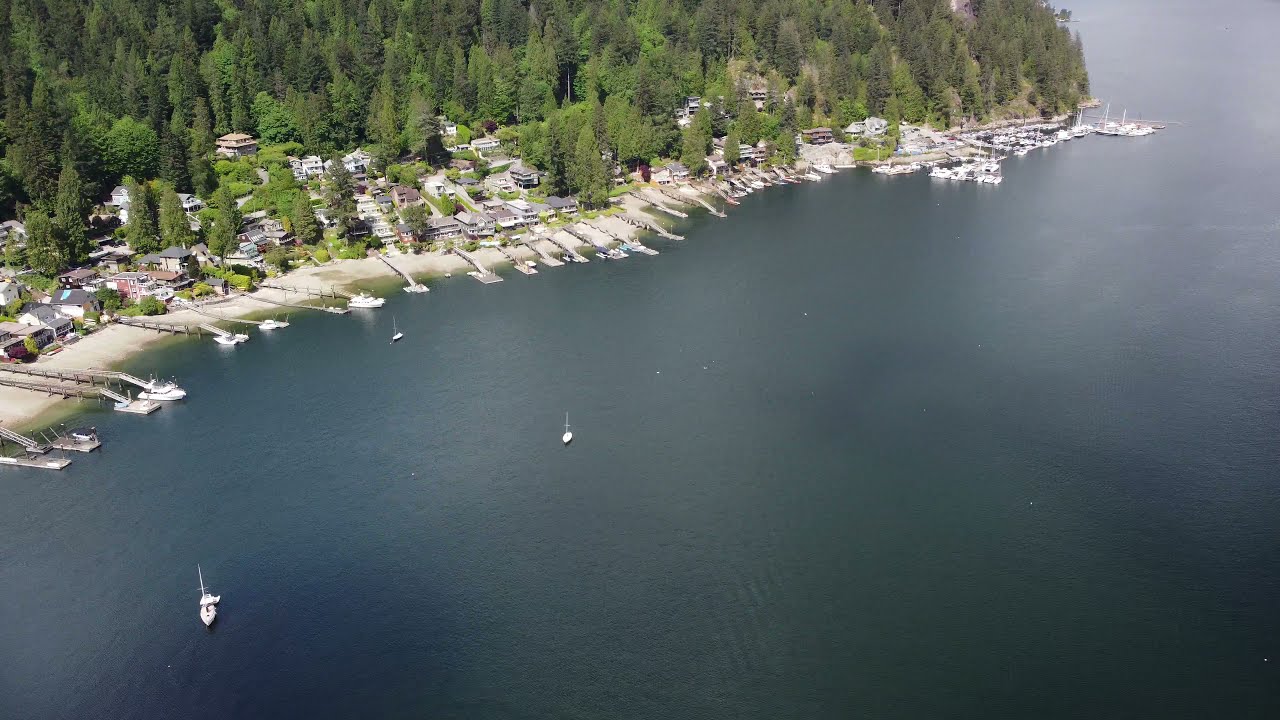The aerial photograph captures a picturesque small town nestled near a large lake, possibly with mountains in the vicinity indicated by the abundance of evergreen and pine trees in the region. The image prominently features a vast expanse of water, likely a large lake rather than an ocean, dominating about 70% of the scene, particularly on the right side and bottom portion of the photograph. The shoreline is dotted with numerous homes and structures, which appear to be cabins or residences designed for tourists or vacationers. These homes are intertwined with a lush, forested landscape rich in green hues. Many docks extend from the shoreline into the lake, providing mooring for various small white boats, some of which are currently navigating the water while others are docked, seemingly ready for use. The serene setting, characterized by the calm, grayish waters of the lake, green trees, and the orderly arrangement of homes, evokes a tranquil, tourist-friendly environment. The top left and top parts of the image are peppered with trees, adding to the densely forested ambiance of the lakeside town.